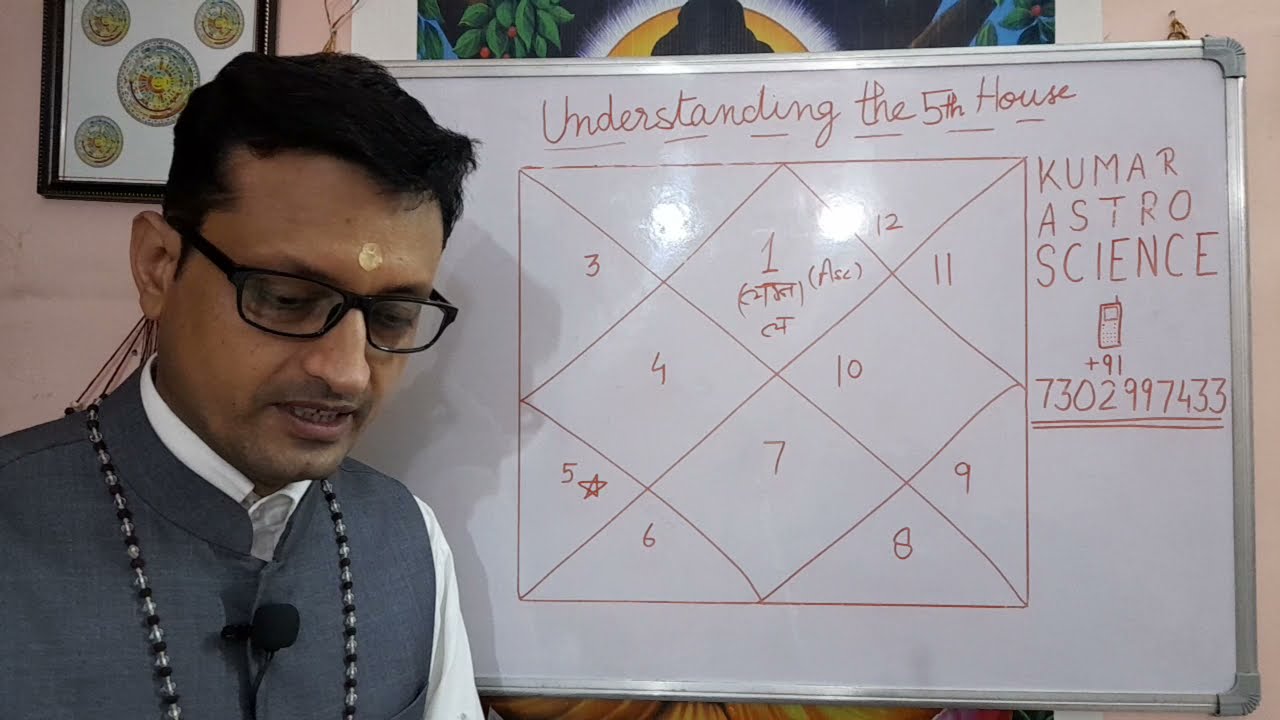The image captures an Indian man, identified by his light brown skin, standing in an indoor setting in front of a whiteboard. He is wearing a white shirt and a gray vest, black-framed glasses, a black and clear bead necklace, a yellow mark on his forehead, and a small black microphone attached to his vest. The man is looking slightly downwards, appearing to speak.

The whiteboard has a detailed diagram and text written on it in dark red marker. The title at the top reads, "Understanding the Fifth House." Below the title is a square divided by a cross with a diamond connecting the four sides. Each section contains numbers: 1 at the top, 4 on the left, 7 at the bottom, and 10 on the right. To the right of the square, the text reads, "Kumar Astro Science," and below it, "plus 91 7302997433."

The background features a cream-colored wall with some artwork, including a religious poster or cloth hanging alongside a picture frame with several seals.